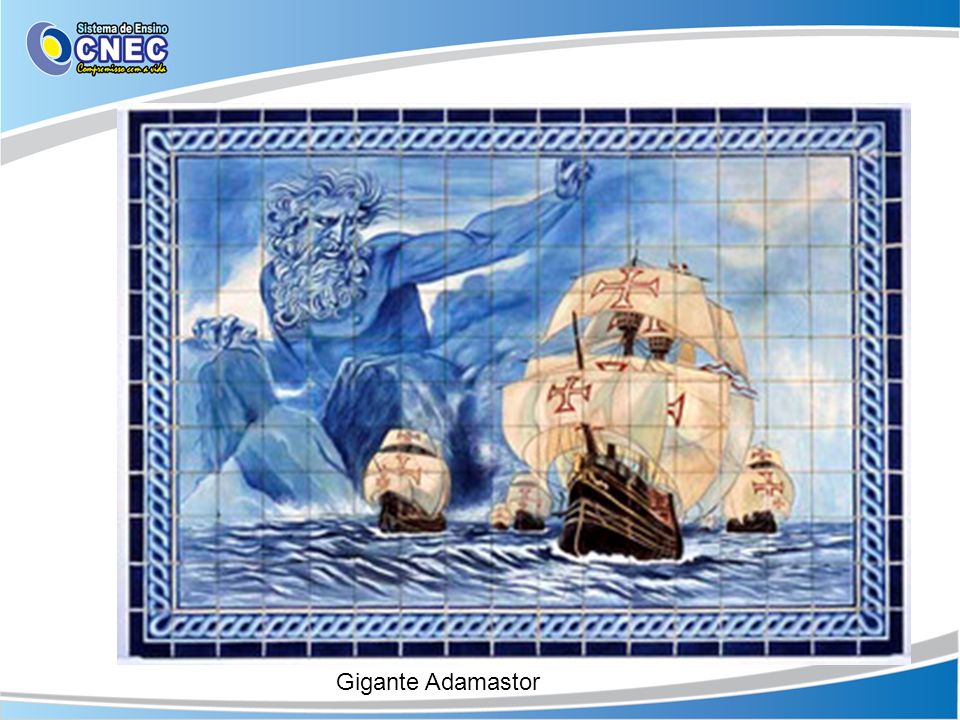The image is a detailed mosaic-style painting of an ocean scene, comprising small, square tiles arranged in a grid format, much like bathroom tile. The border of the image features an intricate pattern: a thin light gray stripe that matches a gradient from light blue to dark blue on the upper and lower edges, highlighted with a decorative blue ribbon shape forming a rectangle. Outside this decorative border, black and white dashed lines create a further framing effect. In the top left corner of the image, the inscription "Sistema de Encino CNEC" is displayed in white letters.

The central scene portrays a turbulent ocean under a stormy, dark blue sky. Dominating the sky and seemingly emerging from both the clouds and the ocean is a colossal blue figure, likely a god resembling Poseidon or another mythological deity. This figure, with an arm raised, appears to be interacting with the setting, either commanding the storm or influencing the waves. Below this divine figure, four brown pirate-style ships with large sails, each marked with a red cross, are caught in the rough sea, their light tan sails fully unfurled as they navigate the waves.

At the bottom of this elaborate seascape, the phrase "Gigante Ademaster" is prominently displayed in black lettering, adding to the grandeur and mythical nature of the scene.